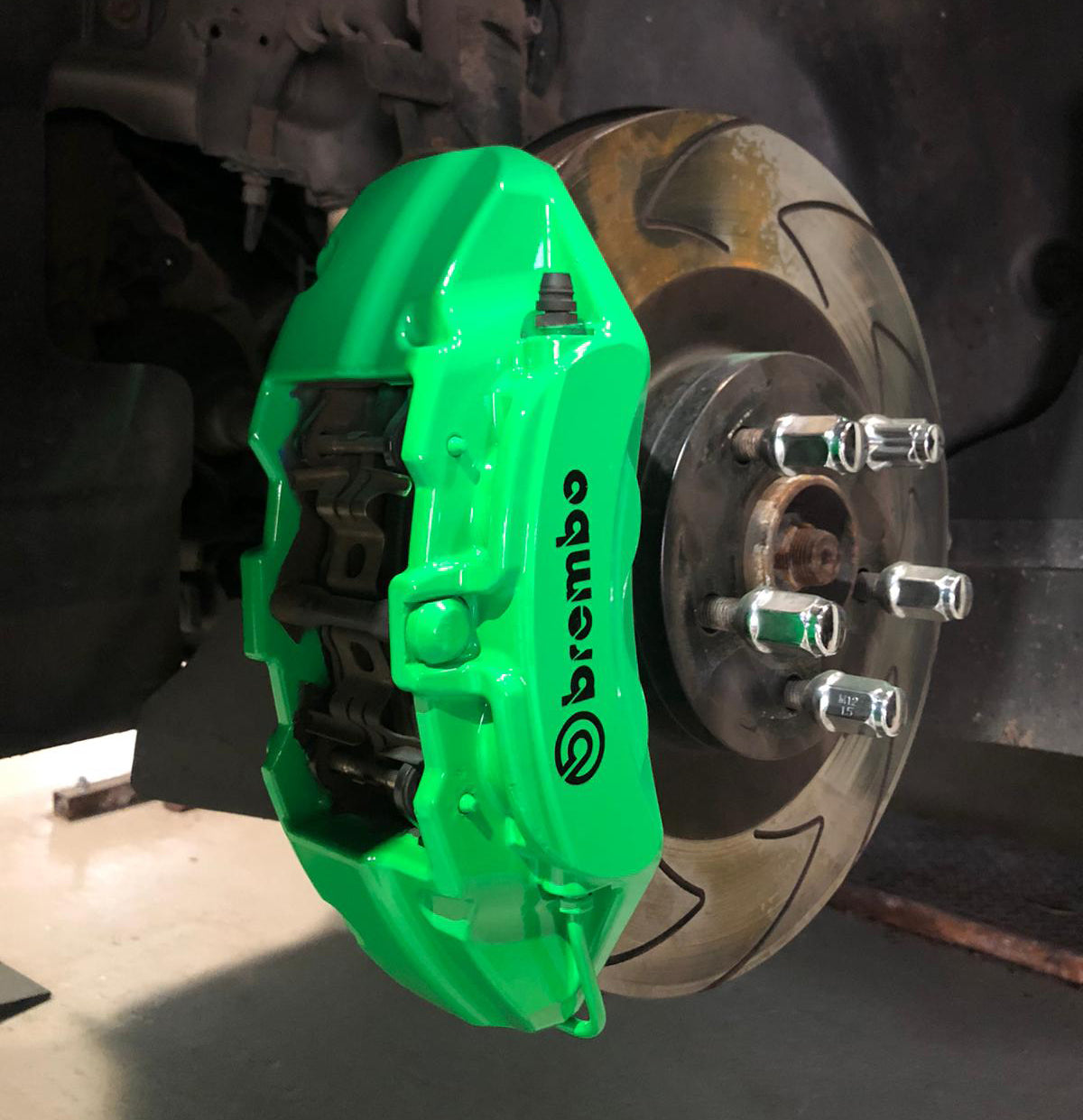In this detailed image, we see the intricate components of a wheel assembly, specifically focusing on the brake disc and brake pad situated within the undercarriage of a car, potentially photographed in a garage setting. The central, circular metal brake disc displays a repeating v-shaped pattern in a gray and brown coloration, while the perimeter of the wheel hub features five silver lug nuts arranged in a circular formation. Prominently attached to this assembly is a bright green brake caliper bracket, inscribed vertically with the word "BREMBO" in bold black letters. This vibrant green component partially encases the brake pad, offering a striking contrast to the metallic tones of the disc. The backdrop hints at the vehicle's internal housing and a glimpse of a concrete garage floor, adding to the industrial and utilitarian feel of the scene.